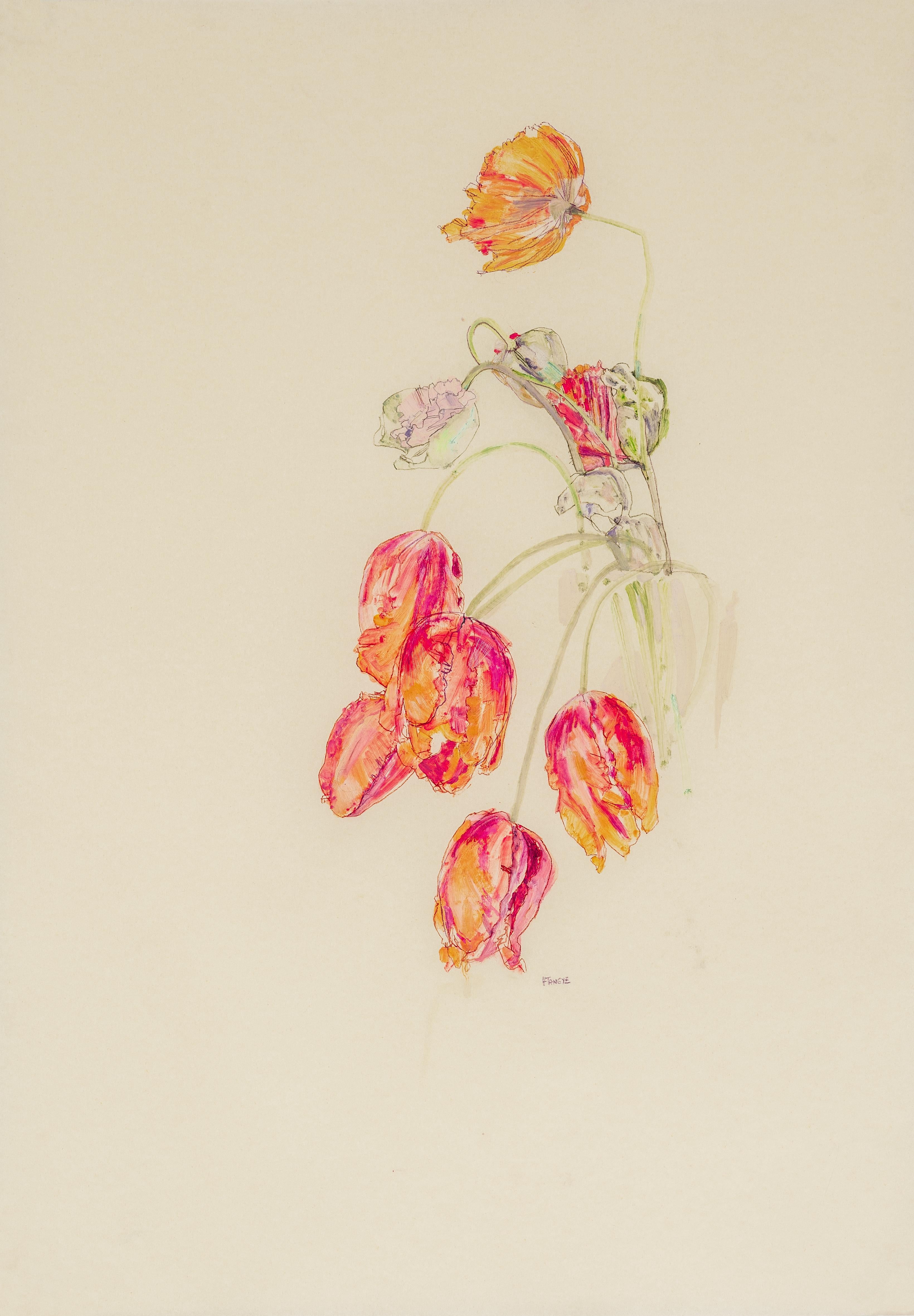This image showcases a delicate watercolor and pen or pencil art piece on an off-white or tannish-pink background. The composition features a cluster of flowers with five prominent tulip-like blooms in the lower section. These tulips have oval-shaped petals that gradient from deep orange to red and are characterized by their bowed, drooping stems. The upper part of the image contains additional flowers: a notably red rose with a green leaf, a pink and green flower, and an orange bloom tinged with red around its edges. The orange flower appears at the top, slightly opened, adding a sense of upward movement in contrast to the drooping flowers below. Overall, the picture captures a moment of fragile elegance, emphasized by thin green stems and sparse foliage. A signature, albeit unclear, is present at the bottom, possibly reading "FL something."